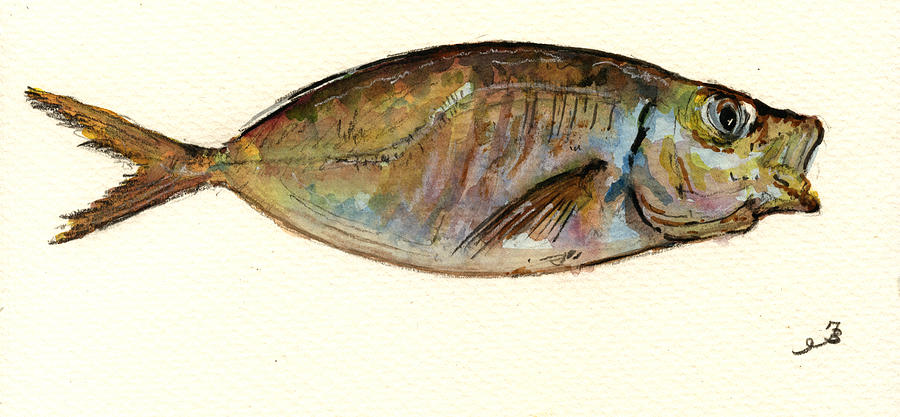This watercolor painting captures a fish, rendered in a horizontal and somewhat narrow orientation. The backdrop is a bright yet subdued yellowish-beige, giving the image a gentle, Zen aesthetic. The fish, which bears a resemblance to a bass or possibly a mackerel, is predominantly brownish-green with accents of green, brown, yellowy-orange, blue, and purplish hues, adding depth and texture to its scales. Its head is slightly more vivid, displaying bluish-gray tones near where it meets the body. The fish has its mouth agape and its single visible eye open, conveying a lifeless, bulging appearance. The creature is notable for its lack of dorsal fins, its smooth, chubby form, and a distinctive V-shaped tail fin, as if a chunk were missing from the typical triangular shape. The textured cream background and visible paper texture enhance the handcrafted feel of the artwork. In the bottom right corner, there is an indecipherable black squiggle, presumably the artist's signature, adding a personal touch to the composition.